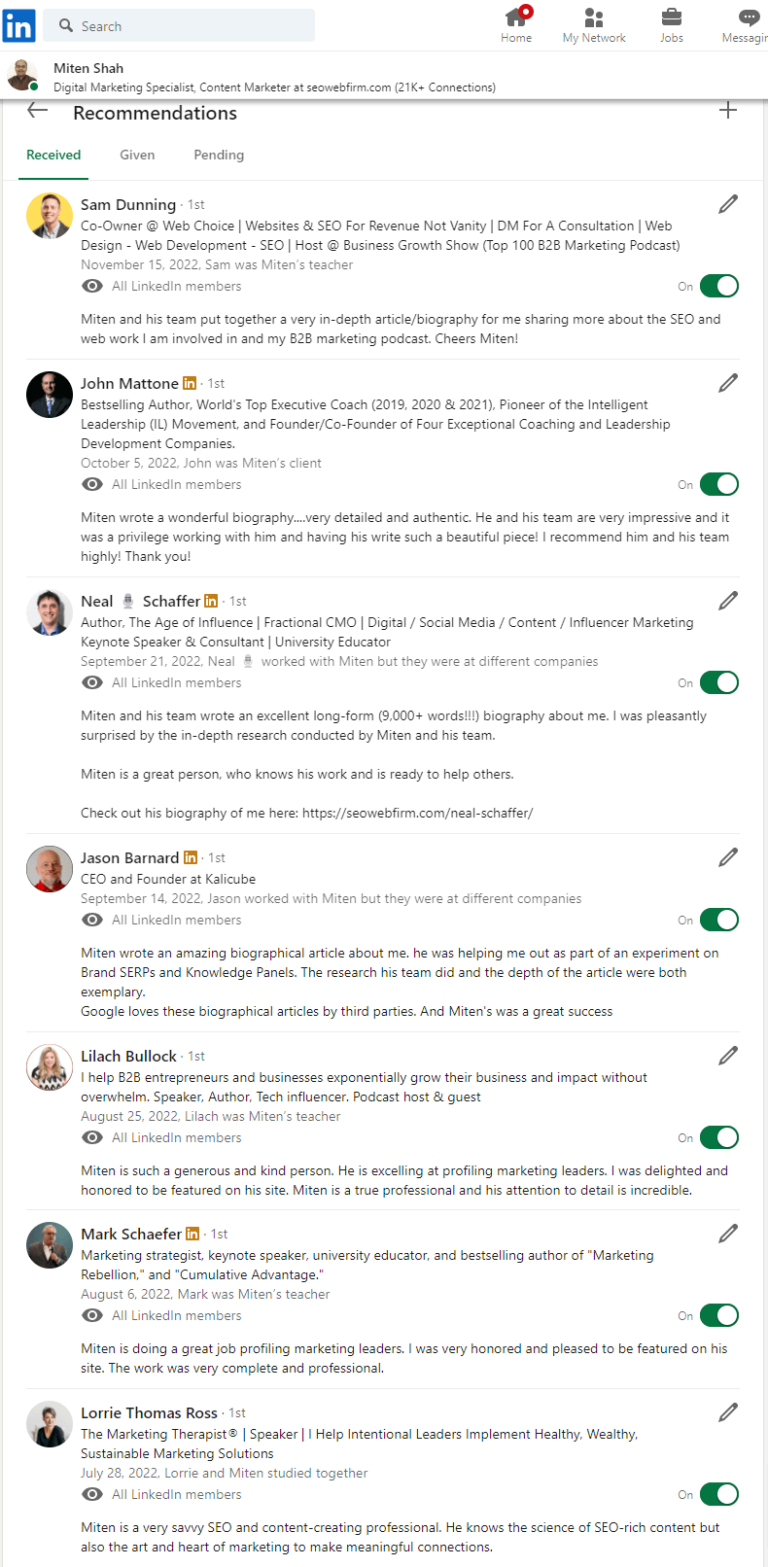This image is a smartphone screenshot displaying the LinkedIn interface against a white background. In the upper left corner, the LinkedIn logo is visible, featuring a blue circle with the lowercase letters "in" in white. On the upper right side, a navigation menu is present, showing icons from left to right: a gray "Home" icon with a red dot containing a white dot, indicating notifications. Next is "My Network," followed by an indistinguishable icon due to small font size, and finally, "Messages" on the far right.

The left side of the screenshot shows the partial profile of the user, though the font is too small to decipher the name. The user's profile photo is small, revealing a person wearing a dark shirt. Below this, the page heading "Recommendations" is prominently displayed. The top recommendation profile features a white man in a white shirt and dark suit jacket, set against a yellow background. The rest of the recommendation text and photos are too tiny to discern clearly.